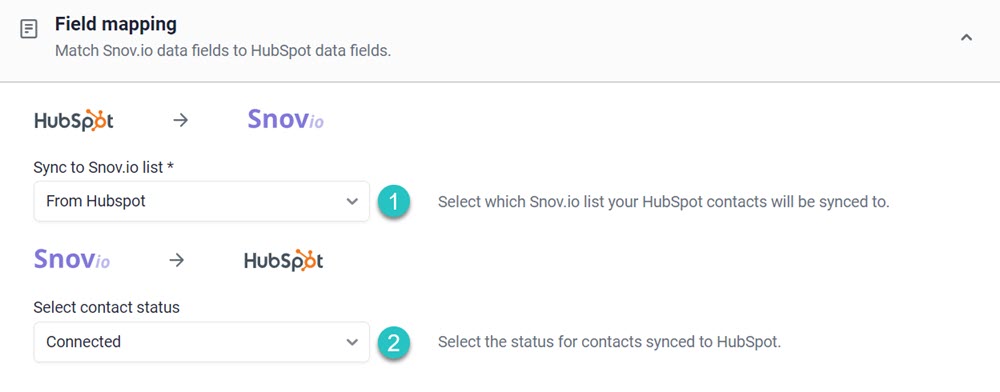The image is titled "Field Mapping" in bold black text at the top. Immediately below, it states: "Match SNOV.IO Data Fields to HubSpot Data Fields." On the left side, there is a small square icon representing text, while on the right side of this section, there is an up arrow.

A horizontal line spans the entire width of the image, separating the top section from the rest of the content. Below this line, the background color lightens to white. The text "HubSpot" is displayed with an arrow pointing right to "SNOV.IO." Beneath this, the text reads, "Sync to SNOV.IO List," accompanied by a drop-down menu labeled "From HubSpot." This menu features a green circle enclosing the number 1, and to its right, it says, "Select which SNOV.IO list your HubSpot contacts will be synced to."

Further down, the text "SNOV.IO" appears with another arrow pointing right to "HubSpot." Below this, it states, "Select Contact Status," followed by a drop-down menu box showing "Connected." This drop-down also has a small arrow for expanding the menu. A green circle with the number 2 is adjacent, and it reads, "Select the status for contacts synced to HubSpot."